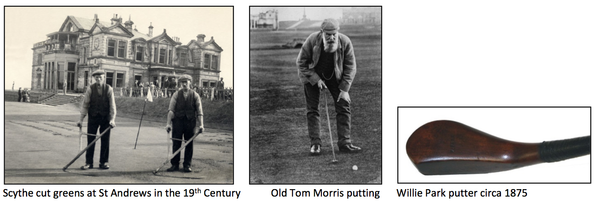In this black-and-white collage, there are three historical photographs side by side, capturing iconic moments in golf history. On the left, an image depicts two men who appear to be identically dressed in caps, vests, shirts, and dark pants, standing in front of what looks like a large clubhouse with dormer windows. These men are holding tools, possibly used for maintaining the greens, with a caption below reading, "Sigh cut greens at St. Andrews in the 19th century." In the middle, an older gentleman, identified as Old Tom Morris, is shown bending over with one hand on his knee and the other holding a golf club, poised to make a putt. The caption for this central image reads, "Old Tom Morris putting." Finally, on the right, a smaller photograph features a wooden golf club known as the "Willie Park Putter, circa 1875," emphasizing its fully wooden design, devoid of any metal components. This carefully curated collage offers a glimpse into the storied past of golf at St. Andrews.